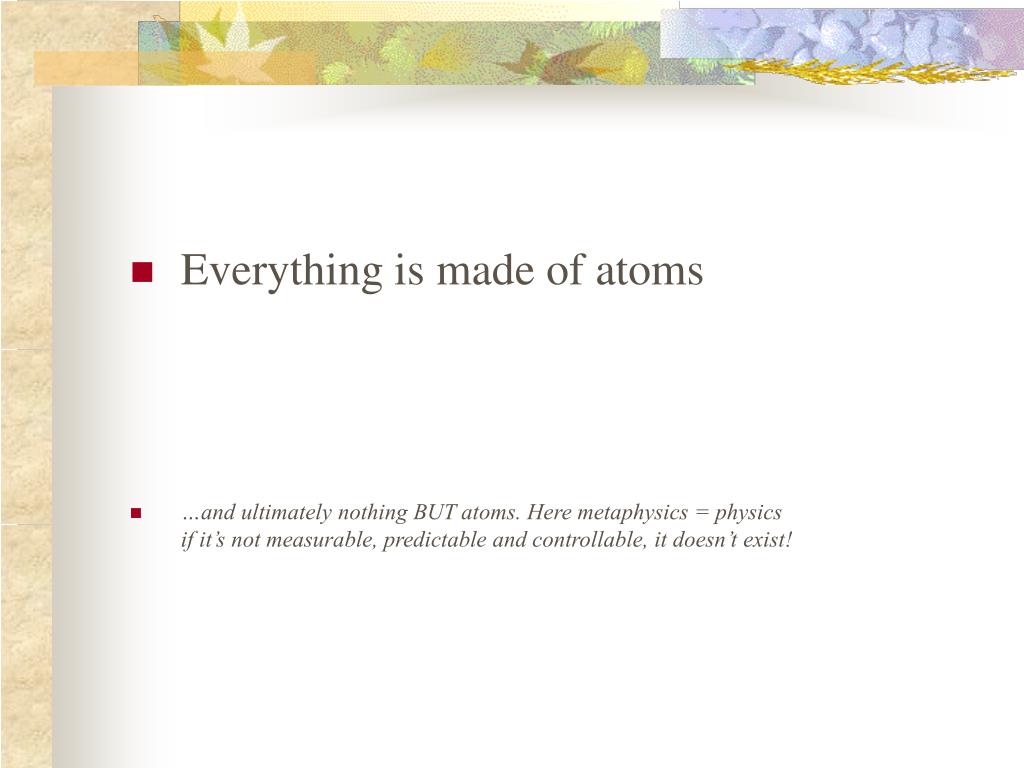The image resembles a PowerPoint slide featuring a primarily white background with a decorative border along the top and left-hand side. The border includes a mix of cream color, green, and off-blue elements with illustrations of wheat, leaves in white and black, and a small pine cone-like or brain matter-like shape. Above the main text area, the leaf and wheat decorations lend a natural, rustic aesthetic.

In the white section, the slide emphasizes important scientific concepts using text formatted with red bullet points. The first red bullet point states, "Everything is made of atoms." A few lines below, another red bullet point continues, "… and ultimately nothing but atoms," with "BUT" capitalized for emphasis. Further down, a smaller black text notes, "Here, metaphysics equals physics. If it's not measurable, predictable, and controllable, it doesn't exist!" This arrangement suggests a hierarchy of importance with bold, red-tinted points leading the narrative about the fundamental nature of reality and the criteria for scientific existence.